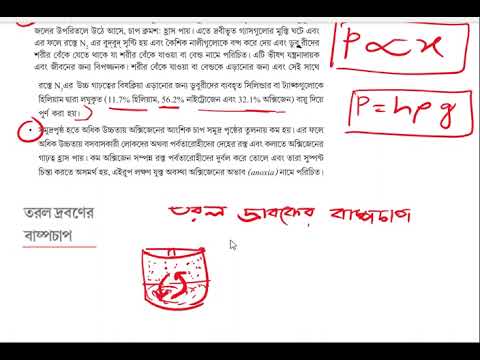The image is a screenshot of what appears to be a page from a textbook, written in an unidentified Asian or possibly Arabic language. The main body of the text consists of black characters on a white background, and includes what might be mathematical or chemical formulas. Several segments of the text are underlined in red ink, with additional red ink notations and annotations in the margins and columns. Noteworthy are the rectangled red-ink notes, which include variables like "P" and equations such as "P = HPG." Toward the bottom of the page, there is a detailed red ink drawing of a container resembling a beaker or cylinder, accompanied by opposing arrows pointing upwards and downwards. The drawing and annotations suggest the page might be detailing some sort of scientific or mathematical problem, with personalized notes and illustrations added for clarification.